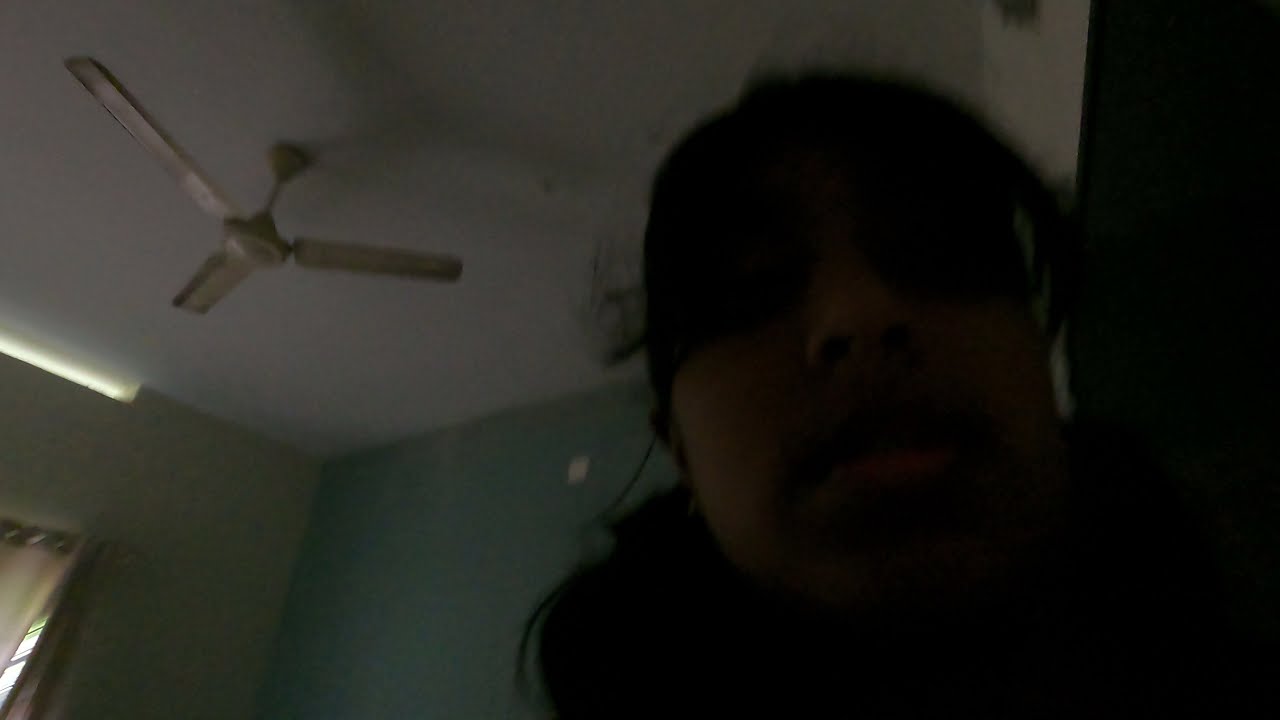In a dimly lit room with the lights off, a dark exposure photograph captures a person standing on the right side of the image. The room features a white ceiling with a three-blade ceiling fan and light green walls. A small segment of a white wall, possibly around a door, is visible to the person's right, while a partially visible window on the left lets in some light, illuminating the otherwise shadowy scene. The wall beside the window has a white patch, potentially an electrical outlet. The person, who may have dark, long hair also resembling a black mustache, stands with indistinct facial features, making it difficult to ascertain their exact appearance. The contrast and blur further obscure the details, though one might guess they are Hispanic or Indian based on subtle hints. The individual might be dressed in dark clothing, blending into the gloom of the photograph.